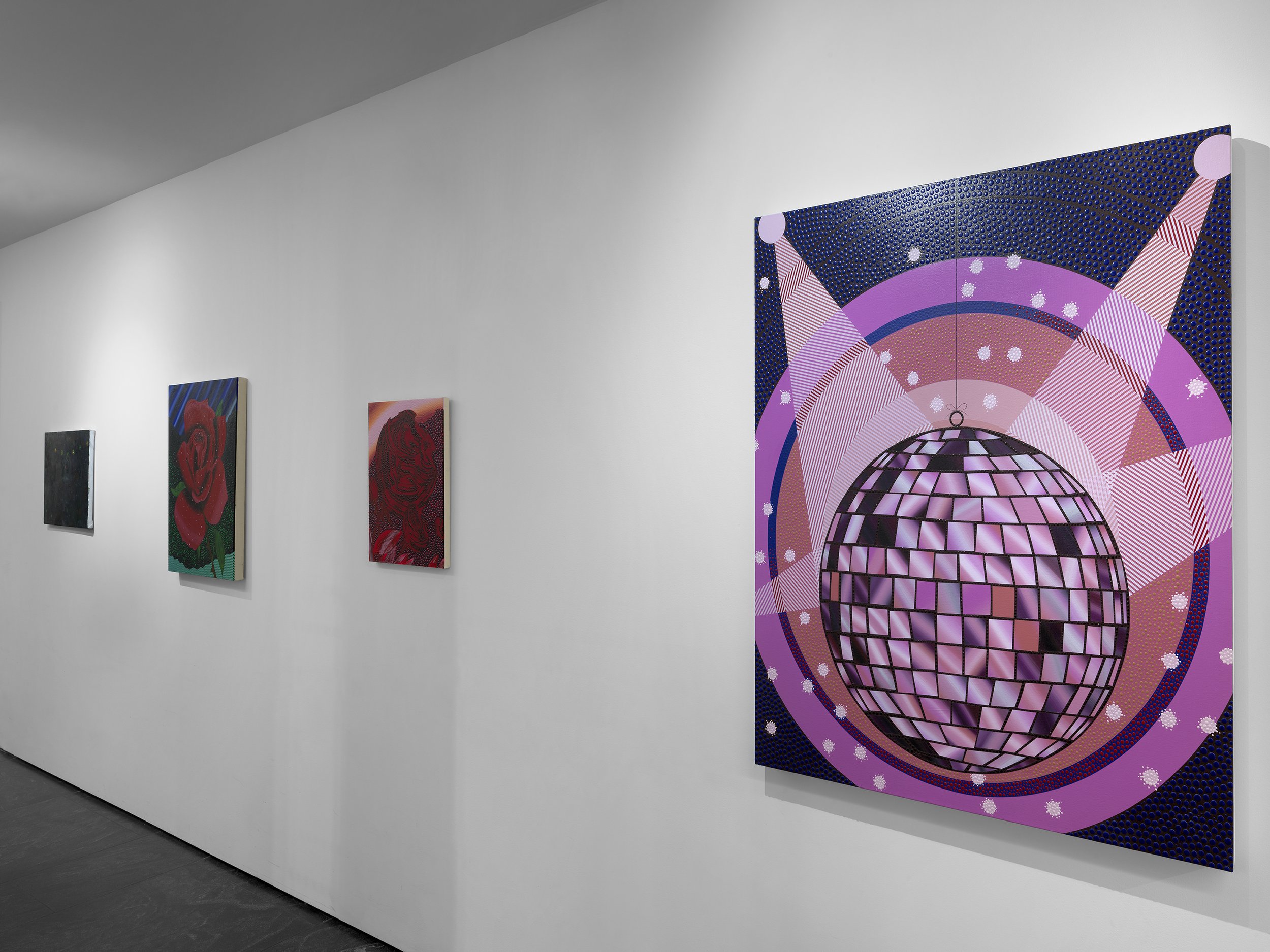This image captures a scene from an art gallery exhibition. The photograph, taken from a slightly diagonal perspective, features a white wall adorned with four distinct paintings. Dominating the right-hand side is the largest painting, depicting a cartoonish disco ball illuminated by spotlights on a predominantly purple and dark blue background. The disco ball is embellished with rings in hues of pink, purple, and black, with white splotches indicating light refraction. To the left of this vibrant piece is a smaller painting of a red rose. Further to the left is a larger artwork showcasing another red rose centered on a background of blue lines and a green base. The final piece, positioned on the far left, is markedly darker, almost entirely black, and obscured in detail. The gallery walls are painted white, adding contrast and focus to the colorful array of art displayed.